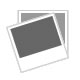A vertically rectangular, animated print of a single-engine, old-fashioned plane in flight against a clear, blue sky. The scene, set outdoors, showcases the plane's propeller in motion and its distinctive white, purple, and orange body with maroon detailing on the wheels and struts. The wings, which are brown, are positioned over the top of the fuselage. The sky-blue background features two green palm fronds extending from the upper right, suggesting the presence of a palm tree just off the edge of the image. The plane's windows are visible, implying room for a few passengers, while a thin black border outlines the top and a thicker border sits below it. The vivid colors and detailed depiction give the image an artistic and nostalgic feel, reminiscent of a vintage aviation scene.